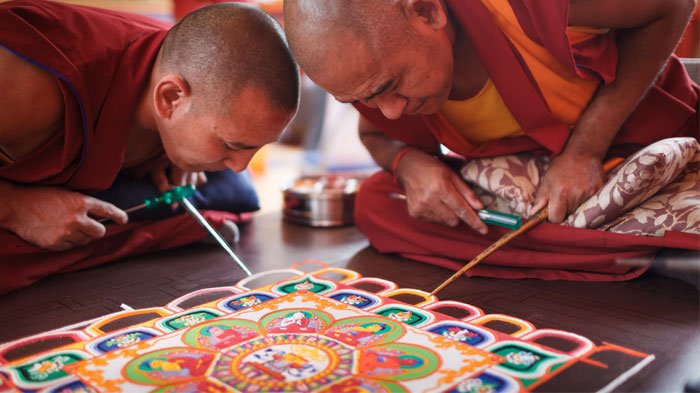In this image, two older Buddhist monks, dressed in maroon and orange robes, are intently working on an intricate, multicolored piece of artwork that spans from the left to right in the center of the image. The monks, who appear to be in their 40s to 60s, are sitting on cushions and leaning close together with their heads almost touching, suggesting a strong sense of collaboration. They are meticulously creating a detailed design with a multitude of colors, including blue, green, red, black, white, orange, and purple, which appears to be a sand sculpture, though it could also be paint or another medium. Each monk holds a stick-like instrument—one brown and the other green/slivered—to manipulate the materials of their artwork. A silver bowl or canister sits between them, likely holding some of their tools or materials. The high quality and detail of the image indicate a recent or modern setting, capturing a moment of focused artistic and possibly spiritual practice.